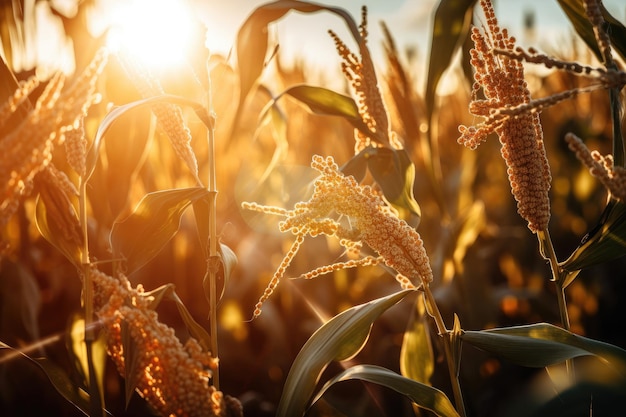The photograph captures a close-up view of an outdoor cornfield or a similar grain crop bathed in sunlight. The image is deeply focused on the foreground, where you can see four distinct corn or grain stalks with light to moderately dark green drooping leaves. The grains are highlighted by the yellow hues reflecting sunlight. In the upper background, the photograph reveals a clear blue sky with patches of clouds, and the glowing presence of the sun in the upper left-hand corner. The field extends into the blurry background, suggesting continuity of similar crops. Scattered throughout the image, particularly on the left-hand side and midsection, are hints of additional plants or flowers, and dots of pink, white, and yellow hues, adding to the detailed texture of the scene. Despite the potential AI generation, the photograph effectively captures the essence and beauty of the agricultural landscape.